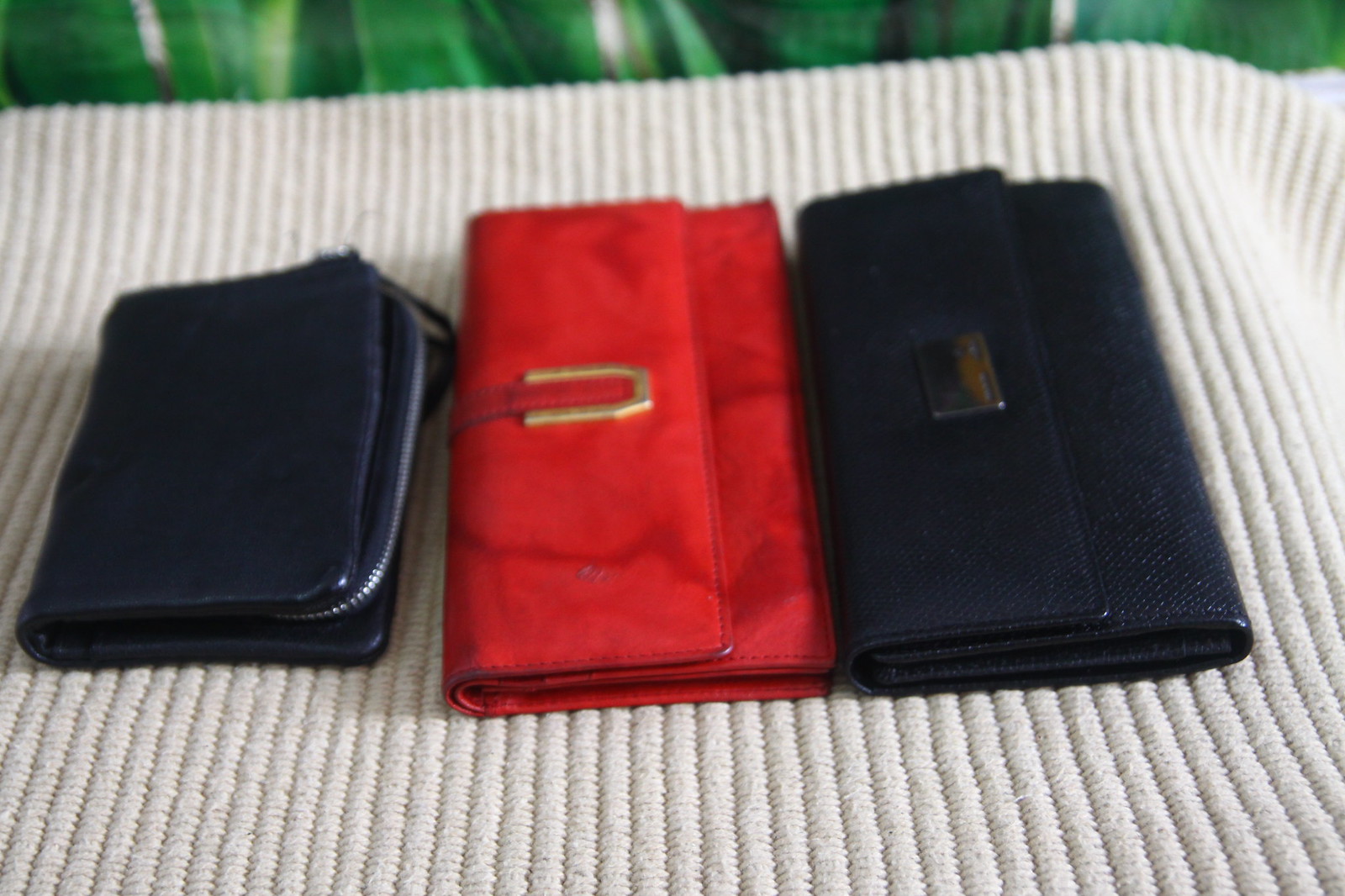This grainy photo captures three distinct wallets positioned vertically on a soft, light beige-brown corded fabric. In the background, long, tall plant leaves stretch across the image, suggesting an indoor setting with artificial light. The wallet on the left is small, black, and features a gray zipper that runs along its rounded side. It appears bulkier despite its smaller size. The middle wallet is red, marked with some faded spots particularly on the corners, and showcases a gold embellishment and clasp on its envelope-style front flap. The wallet on the right is a black leather envelope-style design, complete with a horizontal rectangle logo on the front. Each wallet, differentiated by size, color, and design, is arranged against the textured fabric that provides a subtle striped effect.